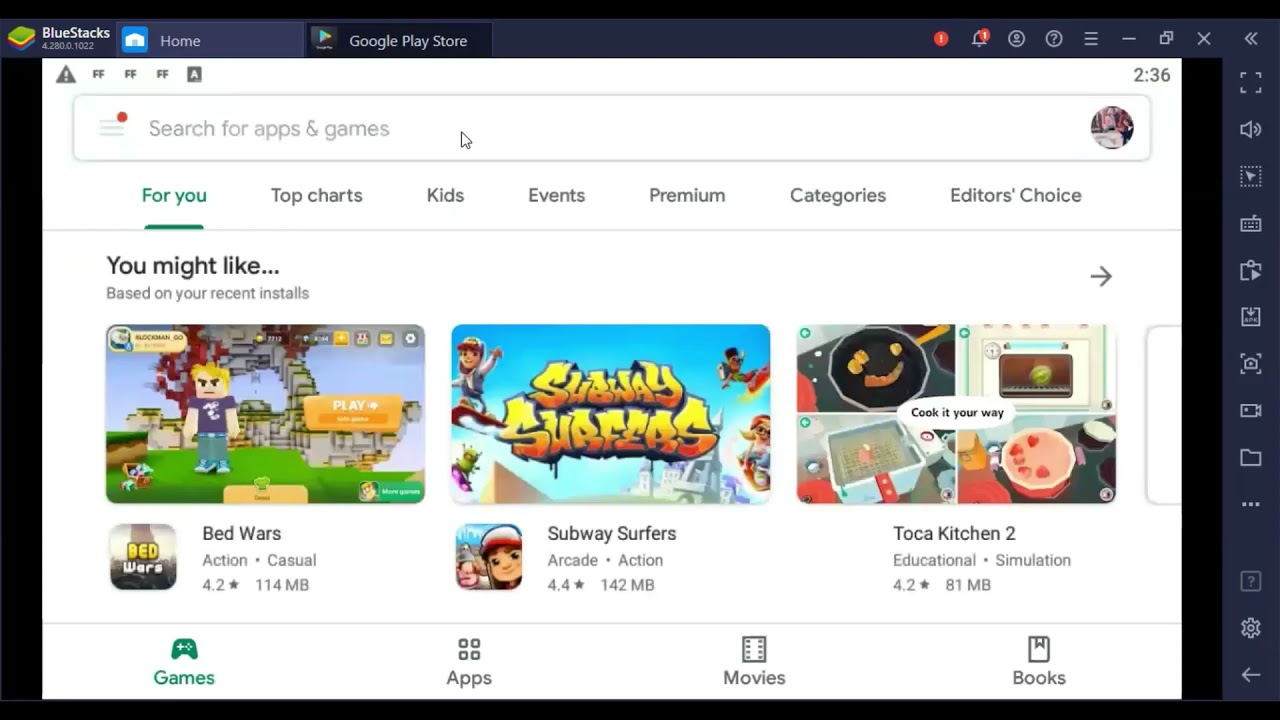This horizontal image appears to be a screenshot taken from a computer, displaying a user interface with a solid, flat black outline. At the top of the screen, there are several tabs labeled "BlueStacks," "Home," and "Google Play Store." In the upper right-hand corner, various icons are visible, including a red circle with an exclamation point, a bell with a notification, a profile image, a question mark, and an options menu represented by three horizontal lines. The window also features the standard minimize, maximize, and close buttons.

Running down the right-hand side of the screen are additional clickable icons. The main section of the screenshot showcases a clean white background, with a search bar at the top that includes a red circle and reads "Search for apps and games." Adjacent to the search bar is a profile circle. Below this search bar, different sections such as "For you," "Top charts," "Kids," "Events," "Premium," "Categories," and "Editor's choice" are listed and highlighted in either teal green or blue.

The area under the heading "You might like, based on your recent installs," suggests apps for download, including "Bed Wars," "Subway Surfers," and "Toka Kitchen 2." At the bottom of the screen, the "Games" section is highlighted in greenish color, with additional options for "Apps," "Movies," and "Books."